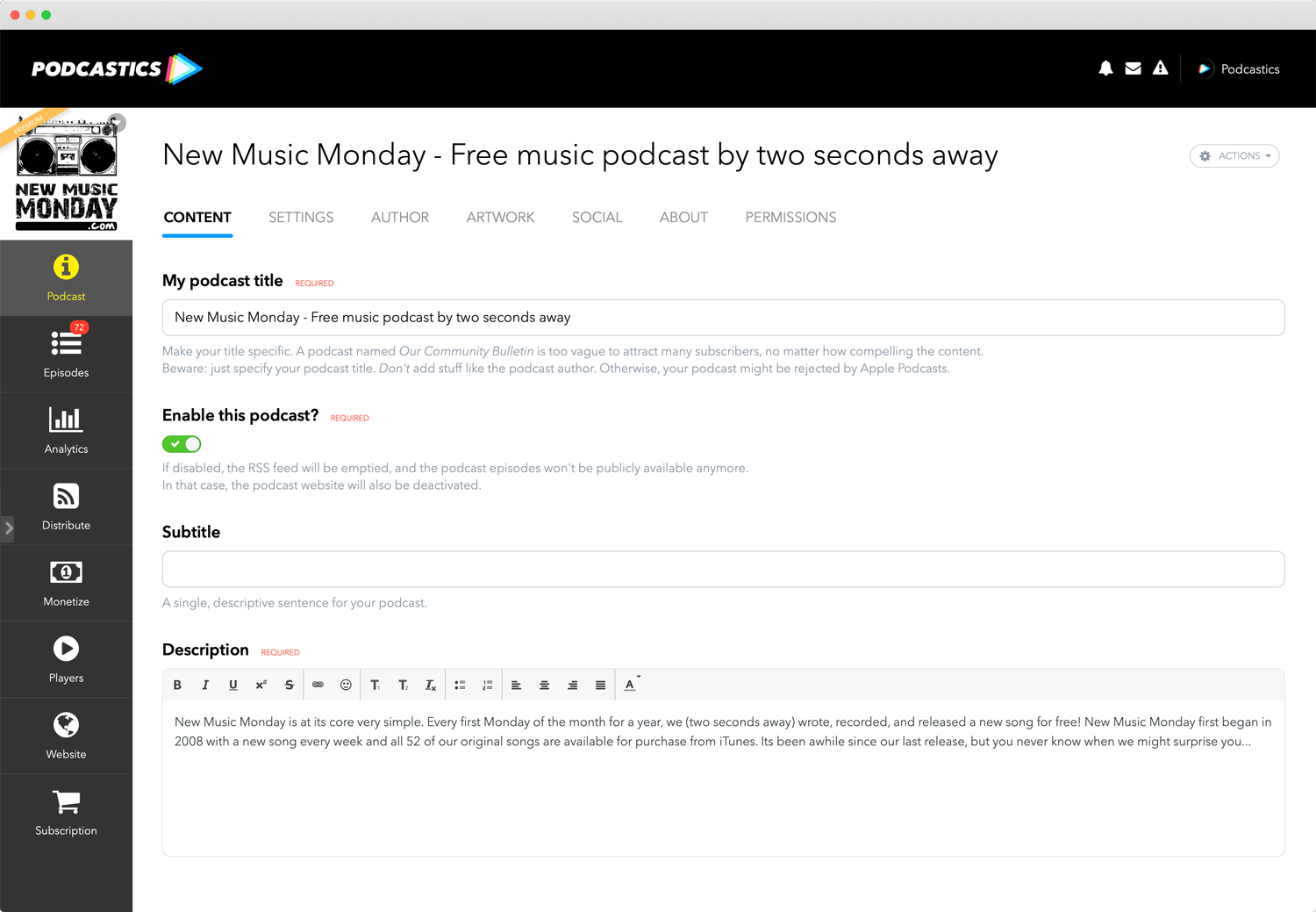The image features a header with a grey border at the top. On the left side of the header, there are three circles in a sequence: red, yellow, and green. On the right side, there are four icons: a notification bell, an envelope, a triangle with an exclamation mark, and the text "PODCASTICS". 

Below the header, there is an image of a boombox with the text "NEW MUSIC MONDAY" over it. To the right of the boombox, in large letters, it states: "NEW MUSIC MONDAY FREE MUSIC PODCAST BY 2 SECONDS AWAY". Under this, several navigation tabs are listed: CONTENT, SETTINGS, AUTHOR, ARTWORKS, SOCIAL, ABOUT, and PERMISSIONS.

Further down, a text box is titled "MY PODCAST TITLE", with a red "required" label next to it. Inside the text box, it says "NEW MUSIC MONDAY FREE MUSIC PODCAST BY 2 SECONDS AWAY". Below this, instructional text reads: "MAKE YOUR TITLE SPECIFIC. A PODCAST NAMED OUR COMMUNITY BULLETIN IS TOO VAGUE TO ATTRACT MANY SUBSCRIBERS, NO MATTER HOW COMPELLING THE CONTENT. BEWARE: JUST SPECIFY YOUR PODCAST TITLE. DON'T ADD STUFF LIKE THE PODCAST AUTHOR, OTHERWISE YOUR PODCAST MIGHT BE REJECTED BY APPLE'S PODCAST."

At the bottom, the text "ENABLE THIS PODCAST" is displayed.